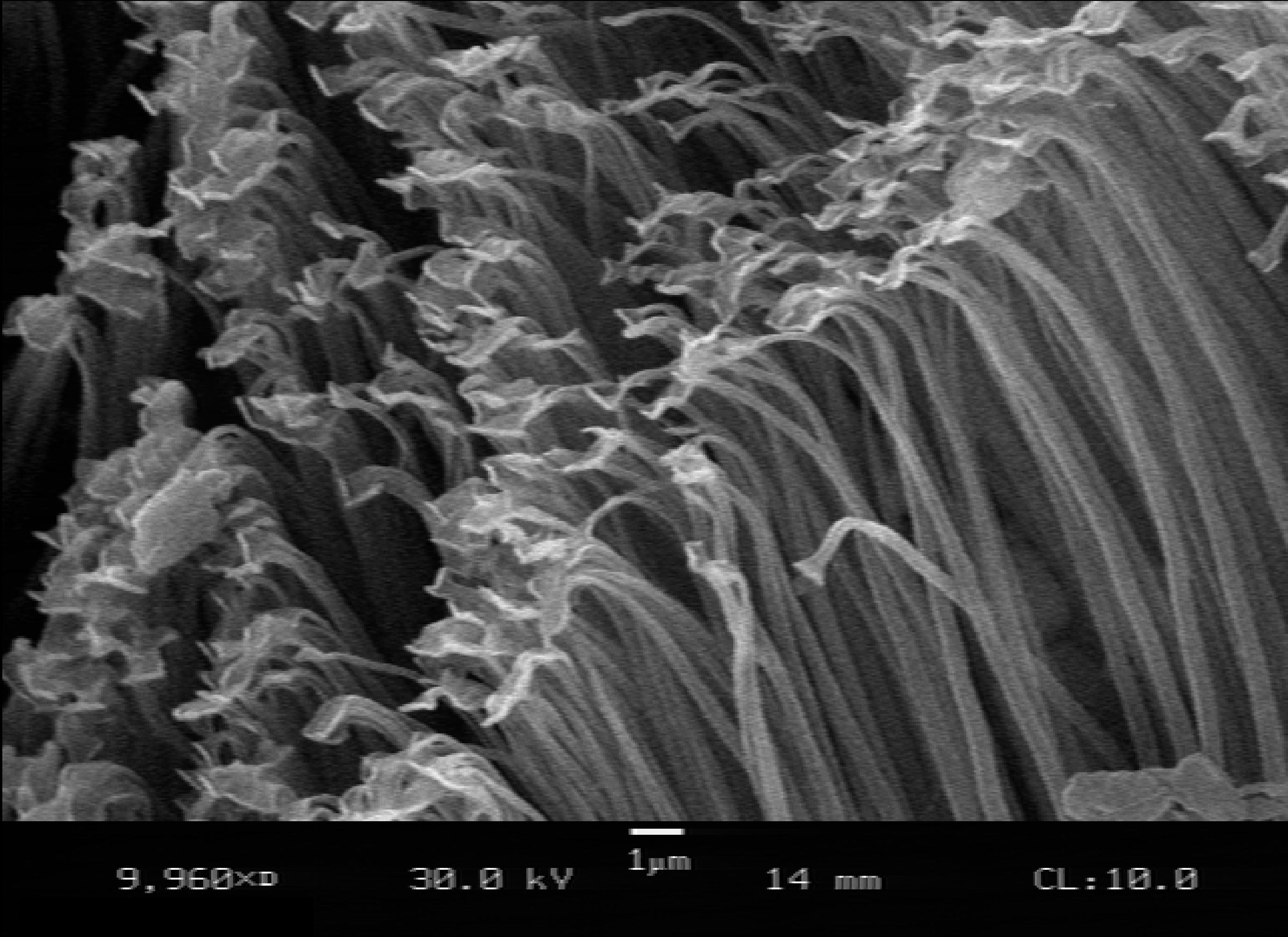This black-and-white image features a striking composition with a prominent black banner at the bottom occupying roughly an eighth of the picture. The banner contains white text that reads: "9.960 times D," "30.0 kV," "1 YM," "14 mm," and on the far right, "CL: 10.0." Above this label section, the majority of the image (about 80%) is dominated by thin, tubular stalks resembling delicate, angel-hair pasta or thin spaghetti. These stalks rise vertically from the black base and curve elegantly at their tops, bending downwards in a cupped shape as if being gently blown from the right side of the image, causing them to bow towards the left. The overall effect is of wispy, white lines against a dark background, creating a dynamic and somewhat mysterious visual experience, possibly generated by electronic waves or a similar process.